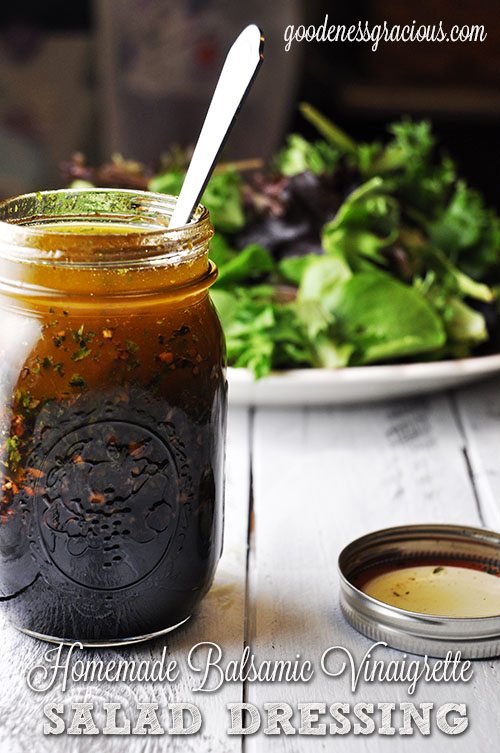In this detailed color photograph set in portrait mode, a mason jar filled with homemade balsamic vinaigrette salad dressing sits prominently in the front left. The dark brown dressing, speckled with beige and black seeds or flecks of spices, has a piece of silverware—likely a spoon—leaning on the inside of the jar. To the right of the jar is its silver lid, placed upside down to reveal traces of vinaigrette inside. The text "homemade balsamic vinaigrette salad dressing" is visible beneath the jar. The background features a softly focused white plate or low bowl filled with mixed salad greens, ranging from light green to dark purple, suggesting a spring mix. The entire setting rests on a wood-planked table. In the top right corner, the script "goodnessgracious.com" adds a final touch to the image.